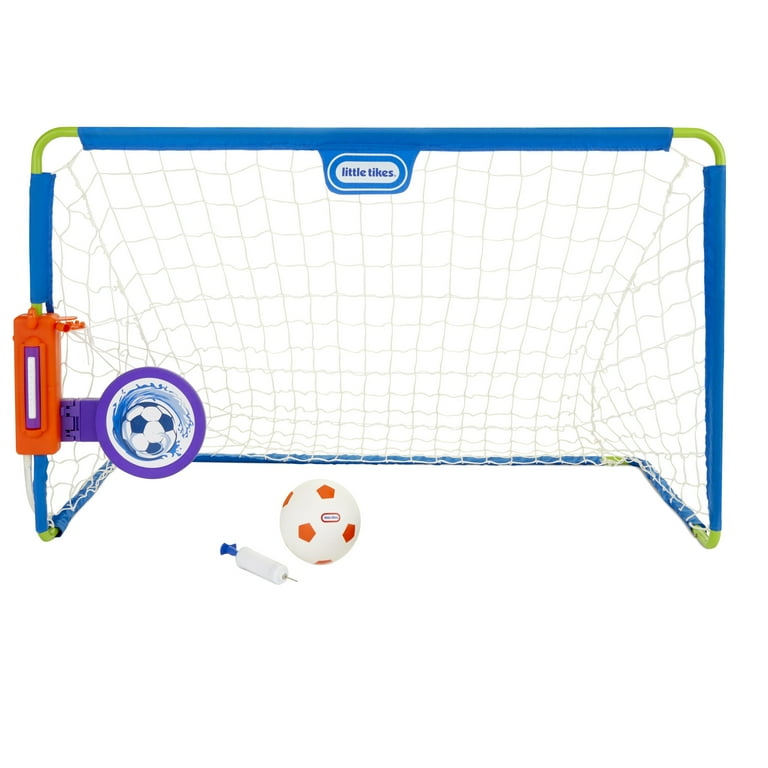This image showcases a Little Tikes soccer goal set designed for young children. The goal features a sturdy frame with a light green metal bar structure covered in blue padding along most parts. The blue padding is prominently visible on the top horizontal bar and the vertical bars on each side, except for the rounded corners at the top, where the green bar is exposed. In the center of the top bar, the branding "Little Tikes" is displayed within a white oval logo. The net of the goal is largely yellow or light green, and it covers nearly the entire goal except for small gaps in the upper left and right corners. Along the left side, there is an intriguing attachment—a red piece connected to the frame that extends into a purple arm ending in a circular target with a soccer ball graphic.

In front of the goal, there is a small soccer ball featuring orange geometric figures and the "Little Tikes" branding. Positioned nearby is a small air pump with a white body and blue handle, possibly for inflating the soccer ball. The entire setup is positioned against a plain white background, highlighting the details and making it suitable for an advertisement.